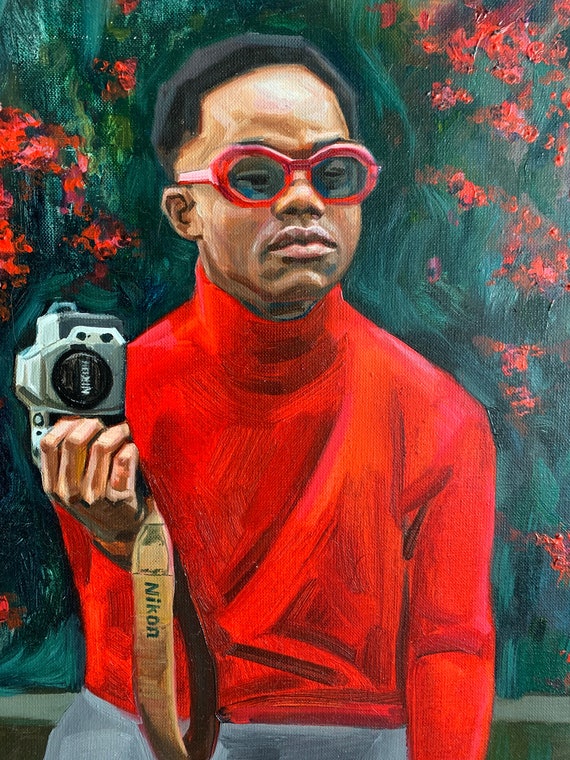This painting portrays a dark-skinned man with a very short afro and black hair, seated and holding a Nikon camera sideways in his right hand, the camera bearing a black lens cover and a beige strap labeled "Nikon." The man dons thick, red-rimmed sunglasses and a red turtleneck long-sleeve shirt, paired with gray pants, and has a sour or slightly frowning expression on his face. The textured background features uneven, sketchy strokes of deep olive green interspersed with red flowers, giving a somewhat blurred and undefined appearance. The combination of these elements suggests a rich, oil painting-like aesthetic that emphasizes the blend of green and red hues with the shades of brown, black, and the vibrant red of the man’s attire.